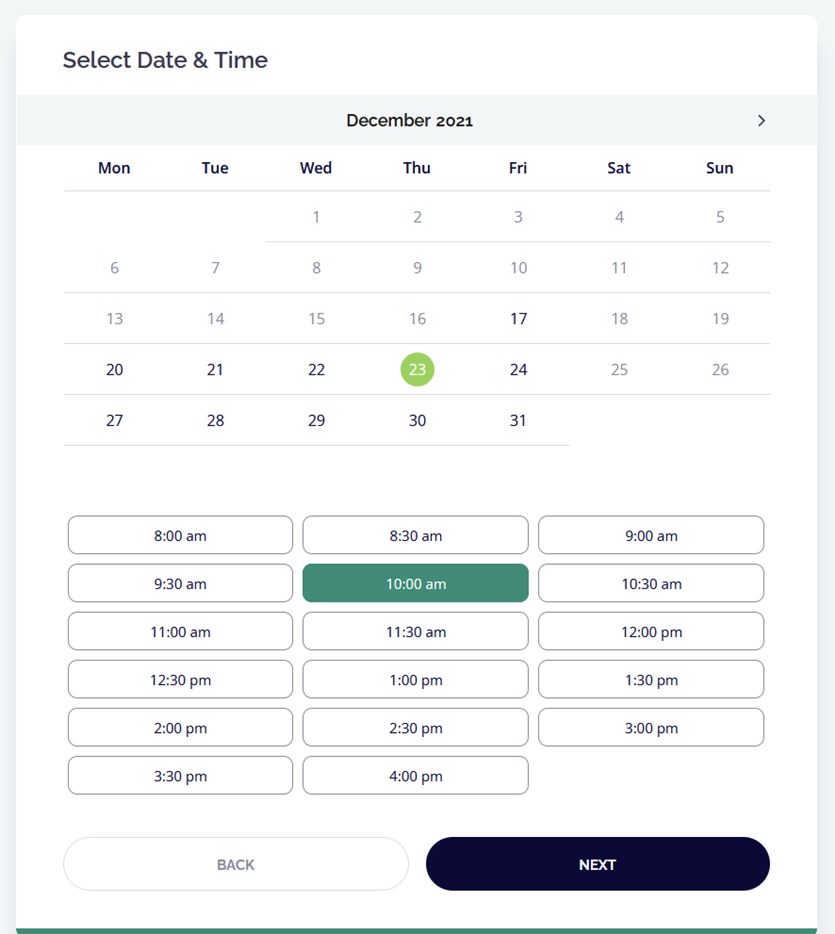The page represents a calendar selection interface with a clean and structured layout. The background is predominantly white, bordered by a thin gray margin at the top and sides, with a narrow green margin running horizontally along the bottom.

At the top of the calendar, the phrase "Select Date & Time" is prominently displayed in large, black font. Directly below this, a light bluish-gray bar spans the width of the page, featuring the text "December 2021" in black font, centered within the bar. Adjacent to this text is a right-facing arrow for advancing the month.

The days of the week are shown from left to right, abbreviated to three-letter formats (Mon, Tue, Wed, Thu, Fri, Sat, Sun). Below this, a nearly full-width gray line demarcates the beginning of the calendar grid. The month starts on Wednesday, with dates presented in light gray until Friday the 17th, which is in black. The pattern continues with some dates in black and others in gray, depending on their significance. Notably, December 23 is highlighted with a green circle containing white text, and several key dates, such as the 20th, 21st, 22nd, 24th, and 27th to 31st, are in black.

The lower half of the page features selectable time slots displayed as buttons. Each button has a white background outlined in gray, with the time written in black. The times begin at 8:00 a.m. on the left and follow a structured pattern: 8:30 a.m., 9:00 a.m., and so forth, until 10:00 a.m., which is uniquely highlighted in green with white text. The sequence continues in this structured fashion until 4:00 p.m.

At the bottom of the page, there are two large buttons. The left button is white with the text "Back" in gray, while the right button is navy blue, featuring the text "Next" in white.

This organized and visually clear layout streamlines the process of selecting a specific date and time.